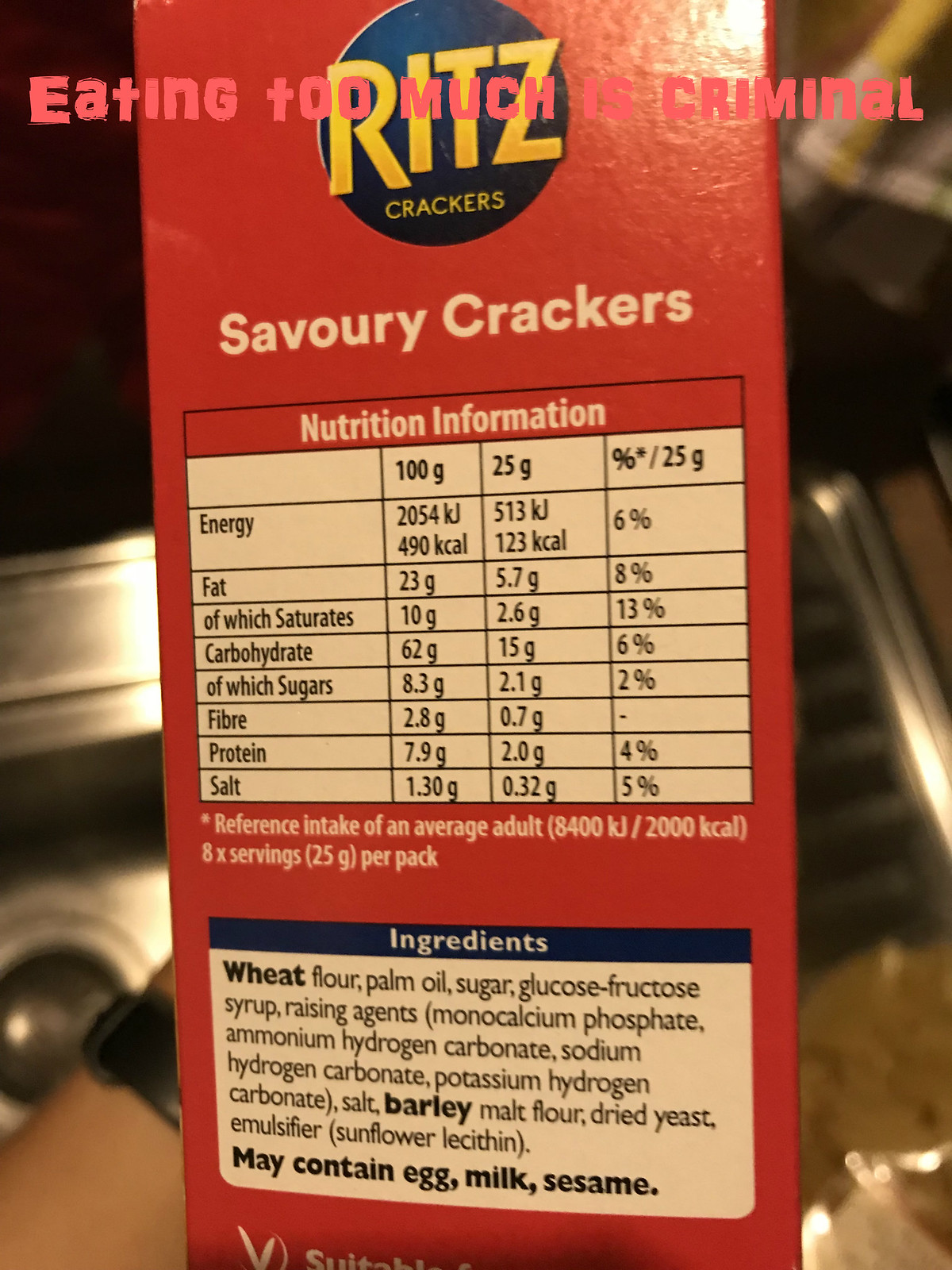This portrait-mode photograph captures the side of a Ritz cracker box being held up by a person wearing a black wristwatch, evident by the visible watch band on their hand. The setting appears to be a kitchen, with various appliances and parts of the kitchen visible in the background, including a bit of beige ground and reflective metal surfaces. At the top of the box, in bold red letters, the phrase "Eating too much is criminal" is prominently displayed. Below this, the familiar Ritz crackers logo sits atop a red background, followed by the label "Savory Crackers" in white lettering. The lower section of the box features a detailed nutritional information chart that lists energy, fat (including saturates), carbohydrate (including sugars), fiber, protein, and salt. Adjacent to the chart is a small rectangular box containing the ingredients list, with certain allergens like egg, milk, and sesame highlighted in bold text. The primary colors visible in the image include red, white, blue, yellow, silver, gray, black, and pink, creating a vibrant and detailed visual representation of the Ritz cracker box.